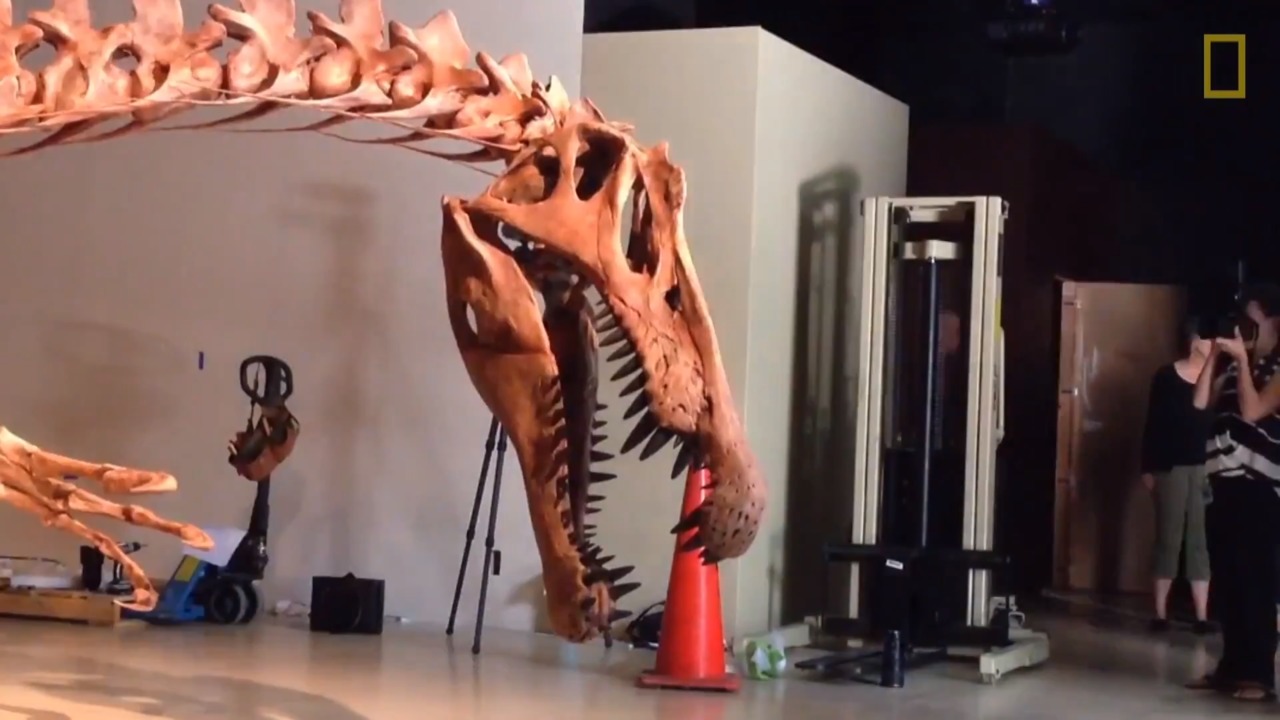This full-color indoor photograph, taken with artificial light, captures a comical and chaotic scene within a studio space, featuring a gigantic dinosaur skeleton as the main subject. The image, which is horizontally rectangular and lacks a specific border or background, includes a digitally added yellow rectangle watermark in the top right corner, reminiscent of the National Geographic logo. Dominating the composition, the dinosaur skeleton's massive head with large, sharp teeth appears to be playfully poised over an orange traffic cone positioned at the bottom center of the frame. The skeleton’s neck and vertebrae are prominently displayed, leading up to the head, with one claw or arm outstretched below. The dinosaur shadow casts underneath, adding depth to the photograph. To the right, two women are engaged in capturing the scene, one holding a camera and the other standing slightly behind her. The background reveals various pieces of photographic equipment, including a tripod, a cart for transporting items, and other mechanical gear, contributing to the overall busy and humorous atmosphere of the image.